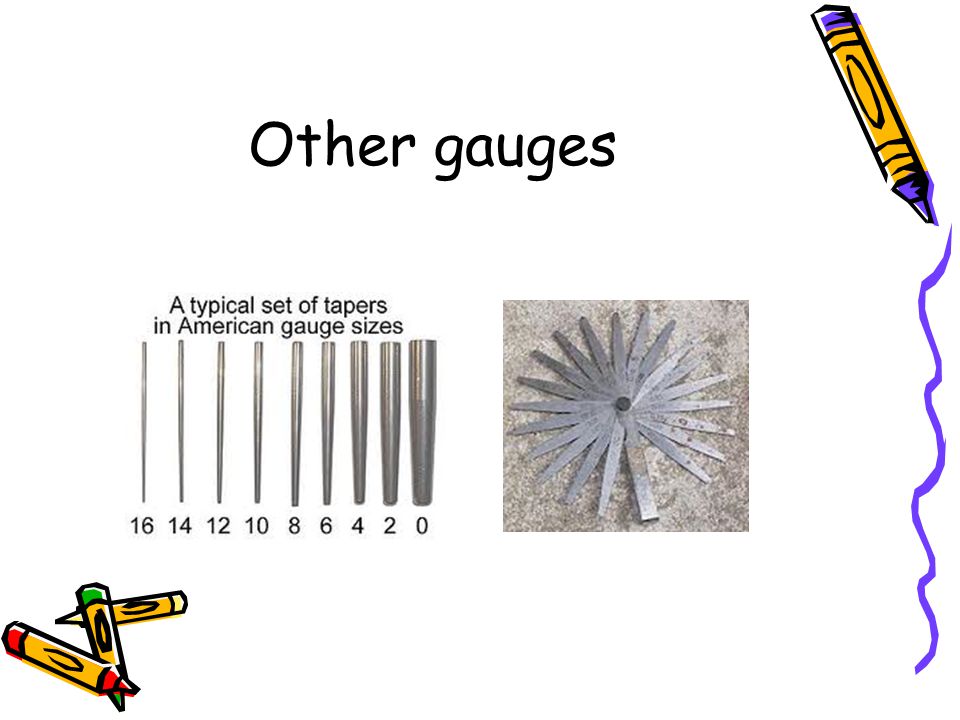This image features a PowerPoint-style slide titled "Other Gages," adorned with graphical elements of crayons. The slide has a whimsical border: a stack of three crayons—red, green, and yellow—decorates the bottom left corner, while a purple crayon draws a vertical line along the right edge. Under the title, the slide is divided into two main sections. On the left side, black text on a white background reads "a typical set of tapers in American gauge sizes," accompanied by an array of nine metallic, pointed objects—the gauges—arranged from thinnest to thickest, labeled with sizes 16, 14, 12, 10, 8, 6, 4, 2, and 0. On the right side, a fanned-out metallic object sits on what appears to be cement. The collage’s color palette includes shades of purple, yellow, red, green, black, white, silver, and gray, blending real objects with digital illustrations.